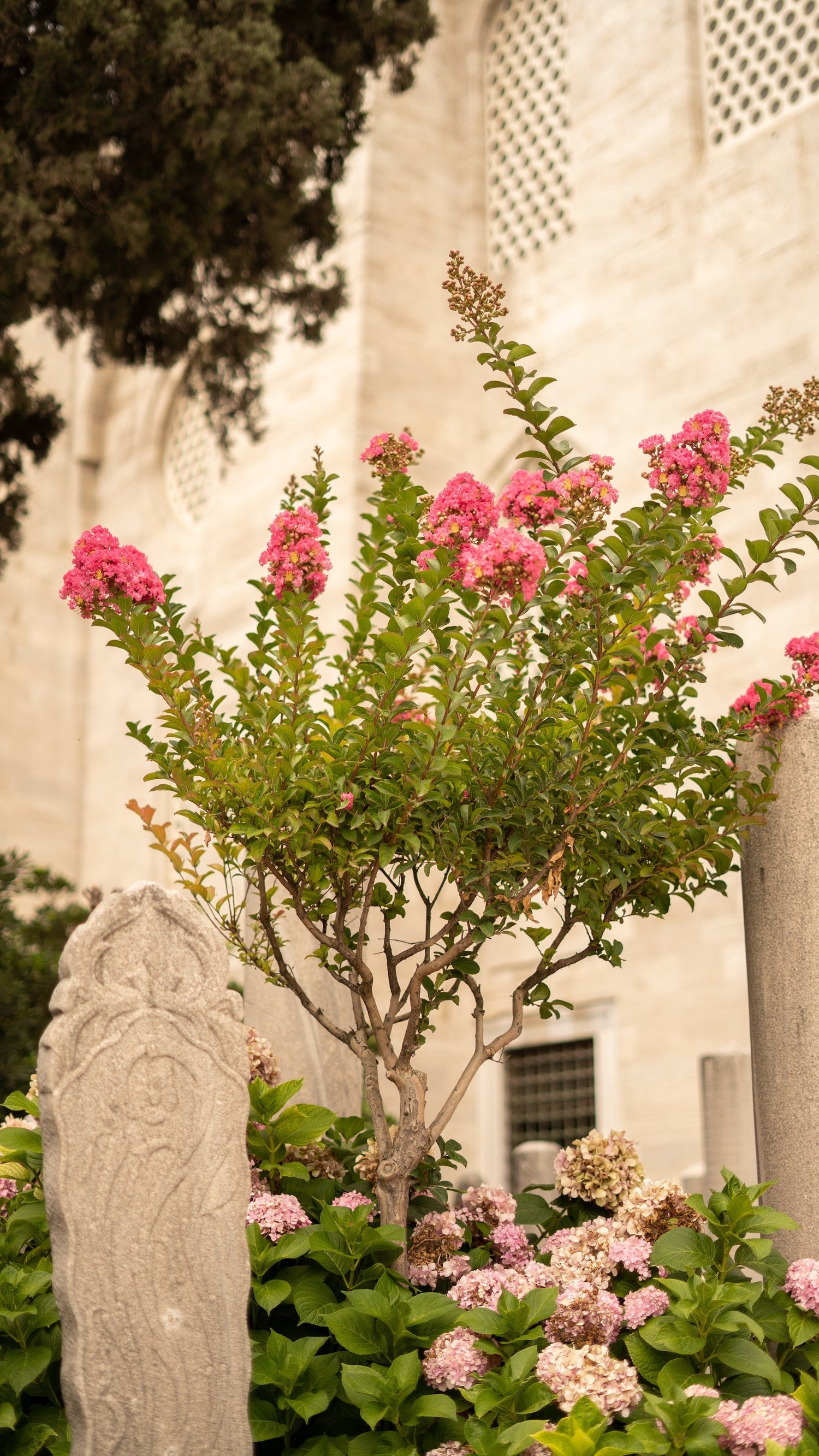This detailed daylight photograph captures a scene outside a white cathedral. In the foreground, a small green bush is adorned with pinkish-white flowers. Flanking this bush, on both the left and right sides, are stone structures that resemble thin tombstones, each with ornate floral carvings. Directly above the bush, another plant with long, slender leaves extends upward, showcasing its small, deep pink flowers at the twig tips. To the left, a tall tree with dark leaves, some protruding into the frame, adds a touch of natural majesty. The cathedral's tan brick face serves as a backdrop, while a beautifully landscaped area enhances the scene with bright pink blooms adorning the greenery. The overall composition highlights the contrast between the delicate flowering plants and the robust architectural elements.